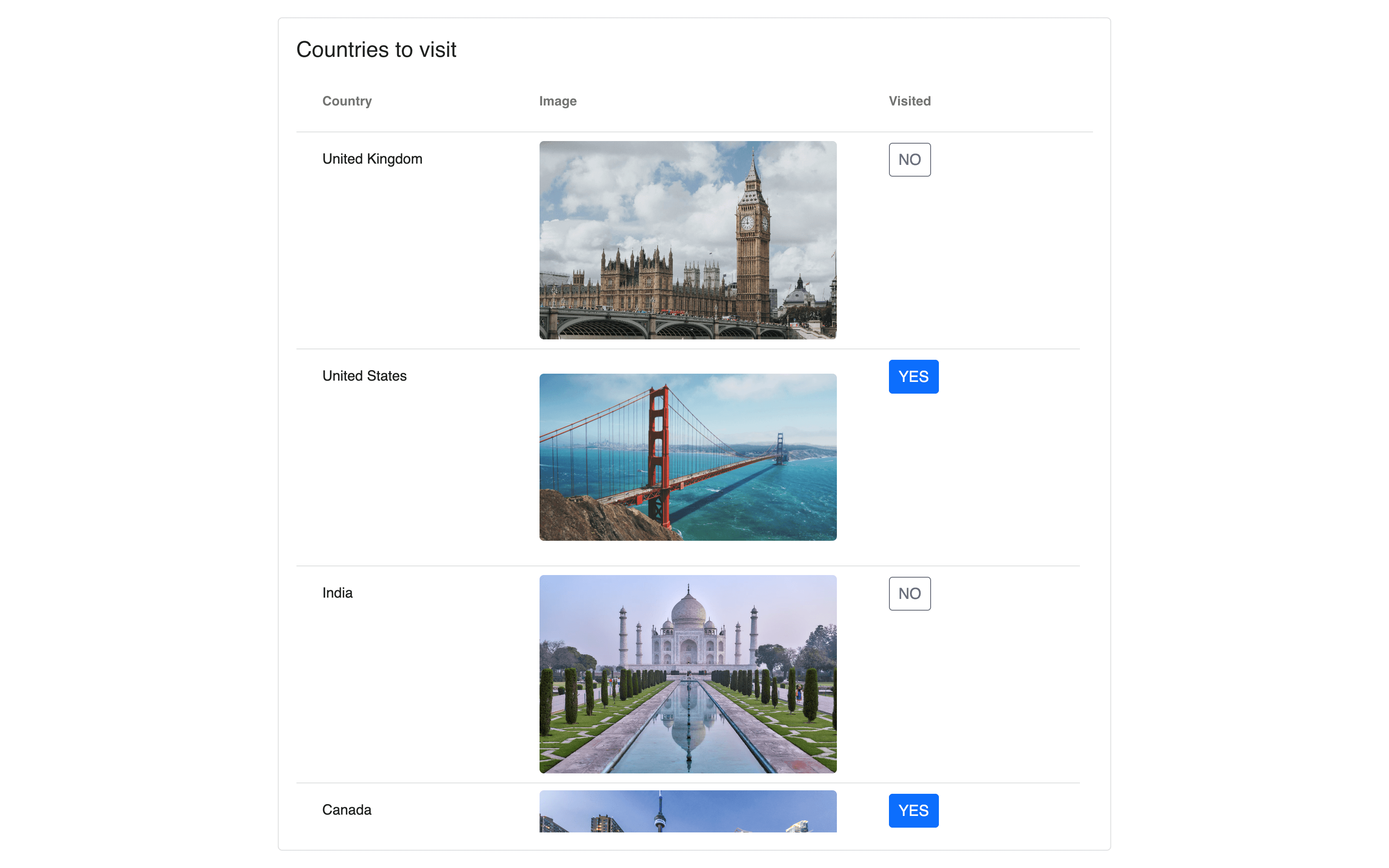This image is a detailed screenshot of a minimalist web page or possibly a list depicting various countries to visit. The background of the web page is white with a clean and simple design. The content is organized into three distinct columns:

- **Left Column**: This column contains the names of different countries, neatly written in text.
- **Middle Column**: Each country name is associated with an image that showcases a notable location or landmark from within the respective country.
- **Right Column**: This column is labeled "Visited" and features status boxes indicating whether the location has been visited. If the box says "no," it is displayed in plain black and white. If it says "yes," the box is blue with white text.

At the very top left of the page, there is a header that reads "Countries to Visit."

Specifically, the list begins with:
1. **United Kingdom**: Accompanied by an image of Big Ben, the visited status is marked as "no."
2. **United States**: Featuring a picture of the Golden Gate Bridge, the visited status is marked as "yes" in a blue box.
3. **India**: Displaying an image of the Taj Mahal, the visited status is marked as "no."
4. **Canada**: Although the image is partially obscured, the visited status for Canada is marked as "yes" in a blue box.

It is implied that there may be additional countries listed beyond the visible portion of the screenshot.